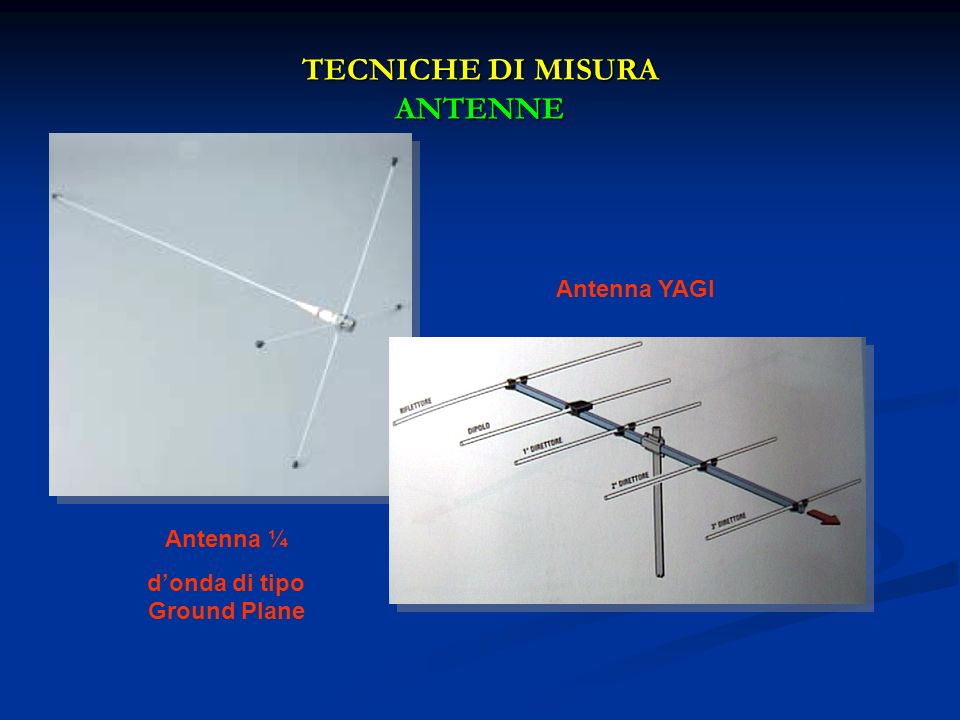The infographic, possibly used for a PowerPoint presentation, features a bold navy blue background that darkens to black at the top. The central focus is on two detailed images of old-fashioned TV antennas. The text at the top of the infographic, written in yellow, reads "Techniche di Misura" followed by "Antenne," indicating it might be Italian. The left image showcases an elongated antenna with a horizontal and vertical rod creating a cross on one end, while the right image presents a more traditional design with multiple rods arranged perpendicularly on a T-bar structure. Descriptions in red text label the left antenna as "Antenna 1-4 Donde Di Tipo Ground Plane" and the right as "Antenna Yagi." Additional small labels are present but difficult to read. The combined elements suggest the infographic is educational, likely illustrating different antenna designs for communication purposes.